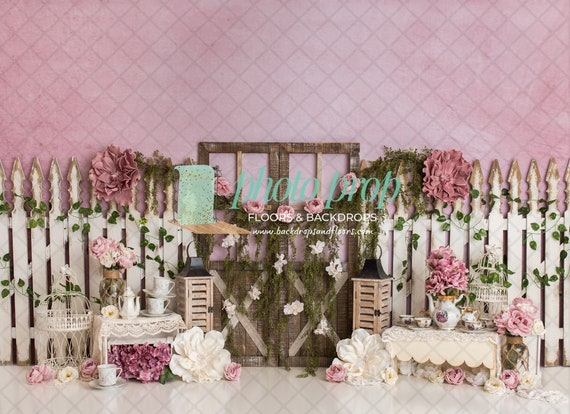The image showcases a charming, boutique-style display set against a pink wall. At the center, a decorative white fence with gold-tipped posts is covered in lush vines and an assortment of pink and white flowers. Nestled within the display is a wooden gate adorned with white flowers. On either side of the fence, small tables draped with baby tablecloths hold teacups, pots of tea, and vases filled with pink flowers, adding to the cutesy aesthetic. The gate features a sign in teal and white text that reads "Photoprop Floors and Backdrops" along with the website "www.backdropsinfloors.com." The entire arrangement is meticulously detailed, with the flowers and vines creating an enchanting, whimsical atmosphere.